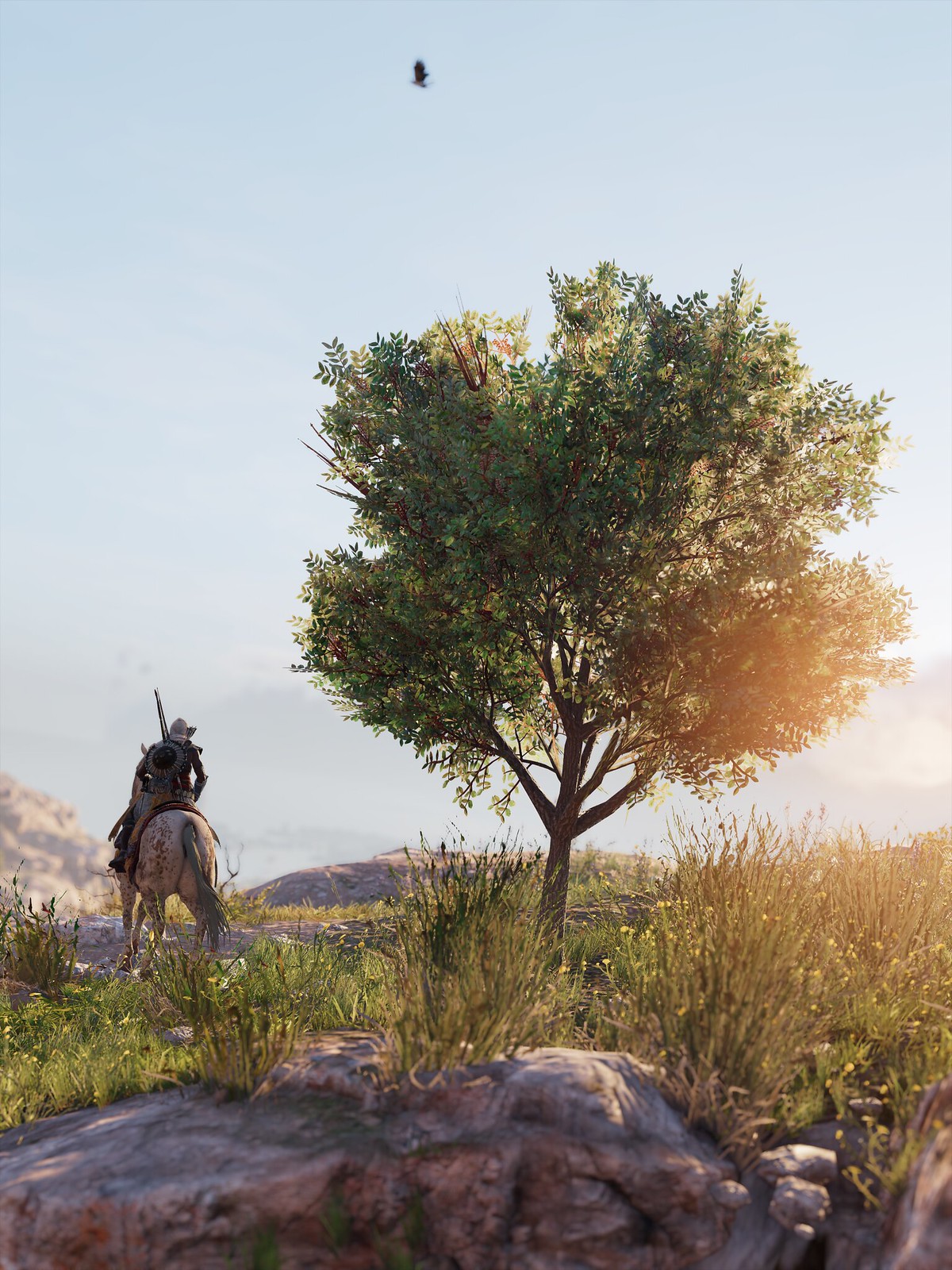This captivating image, likely AI-generated due to its surreal elements, portrays a serene yet stark landscape resembling a remote, arid desert or a dry, mountainous area. Central to the scene is an impressively tall tree with a robust brown trunk, adorned with abundant green foliage that resembles the dense clusters of a broccoli head. Interspersed among the leaves, vibrant red fruits or other round objects add a striking contrast to the greenery. 

In the foreground, a distinct tannish-red rock formation stands out, surrounded by patches of dry, brownish-green grass, characteristic of an austere, parched ecosystem. To the left of the image, a man is seen atop a white horse speckled with brown spots. The man is equipped with a backpack and possibly armor, and noticeably, he appears to be carrying a gun. The composition and details, while vivid and richly textured, lend a fantastical quality to the scene, reinforcing the impression of it being an AI-crafted visual.